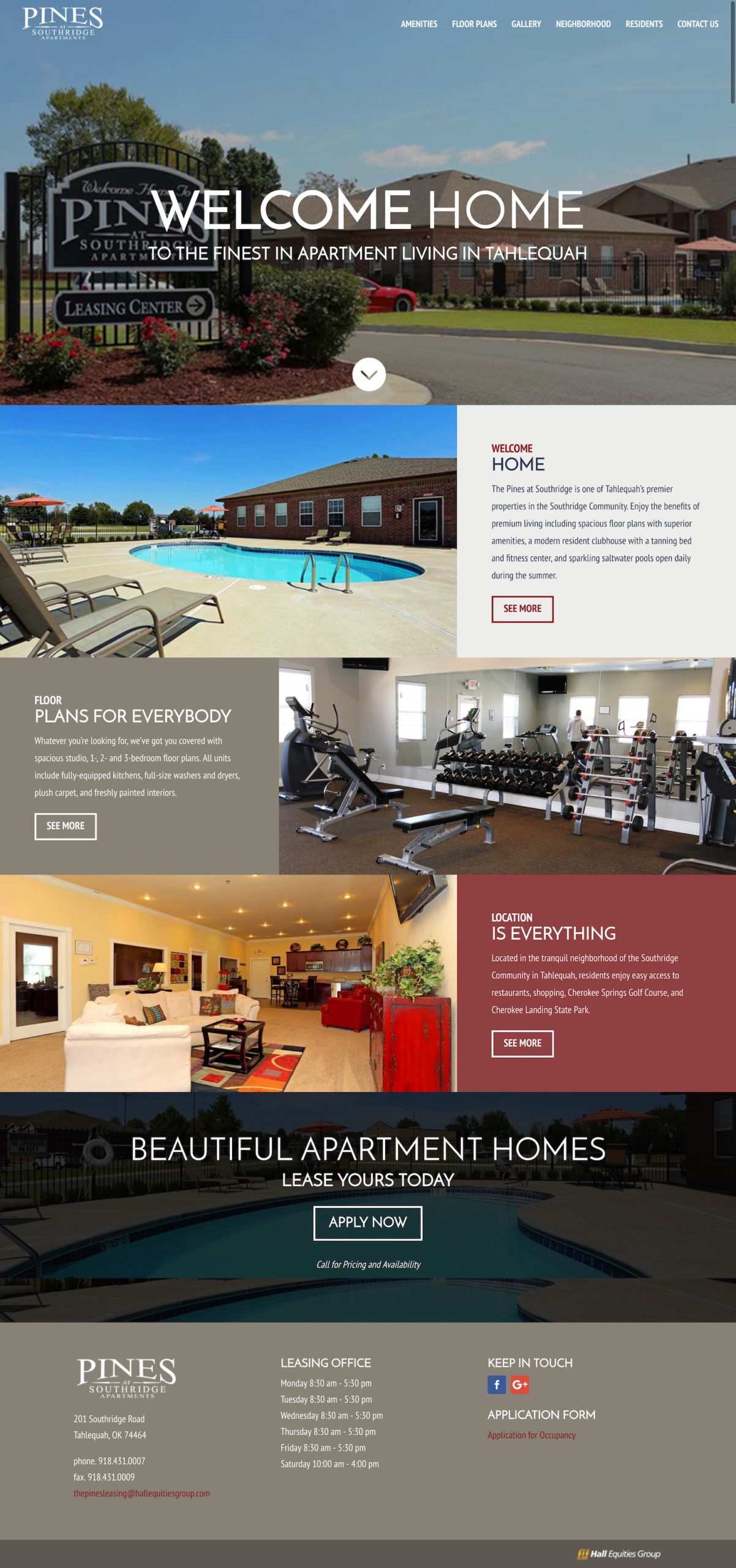This image showcases a low-resolution mock-up of a website for an apartment complex or multiple complexes within a gated community. The banner at the top warmly greets visitors with the phrase "Welcome Home" in crisp white text. Dominating the visual is a picturesque scene of the gated community, showcasing a welcoming sign, elegant single-floor houses resembling townhomes, and lush green lawns. The headline underneath reads, "The Finest Apartment Living in Temecula."

The body of the webpage features alternating blocks of text and images, presenting various amenities available within the complex. While the text on these banners is mostly illegible due to the resolution, they are color-coded—one is white, another dark gray, and yet another a burgundy reddish hue—each highlighting different aspects of the apartments. These sections are complemented by attractive promotional photos, including a well-maintained pool, a fully-equipped exercise area, and a stylish lounge space.

Toward the bottom of the page, a call-to-action boldly proclaims, "Beautiful Apartment Home – Lease Yours Today, Apply Now," accompanied by an image of a luxurious-looking pool, reinforcing the upscale nature of the community. The final gray banner displays vital information about the apartment complex in white text. This section also includes clickable elements, presumably email addresses, in red, and several social media icons, with Facebook being the only one clearly identifiable.